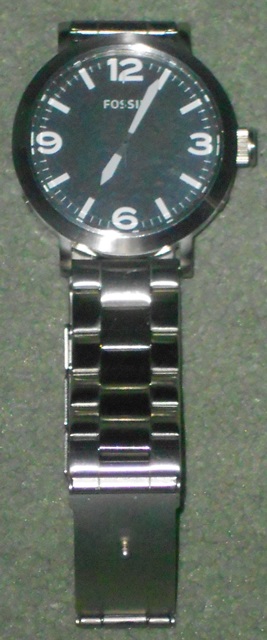This is a photograph of a silver men's Fossil watch taken from above, displayed on a medium grayish-greenish background that adds a monochromatic feel to the image. The watch, featuring a large round face, is positioned with part of its wristband at the bottom. The silver metallic band, composed of adjustable links, lays open with the clasp visible.

The face of the watch is predominantly black or dark blue, with prominent white numerals marking 12, 3, 6, and 9 o'clock, while the remaining hours are denoted by simple white slash marks. The brand name "Fossil" is clearly visible below the 12. The watch hands are white, with the hour hand pointing to 7 and the minute hand to 5, indicating the time as almost 7:05. A silver winder knob is seen on the right side of the bezel. Notably, there is a reflection on the lower part of the watch face, suggesting a flash was used when taking the picture. Overall, the colors in the image are a blend of gray, silver, white, and black, contributing to its understated, classic look.